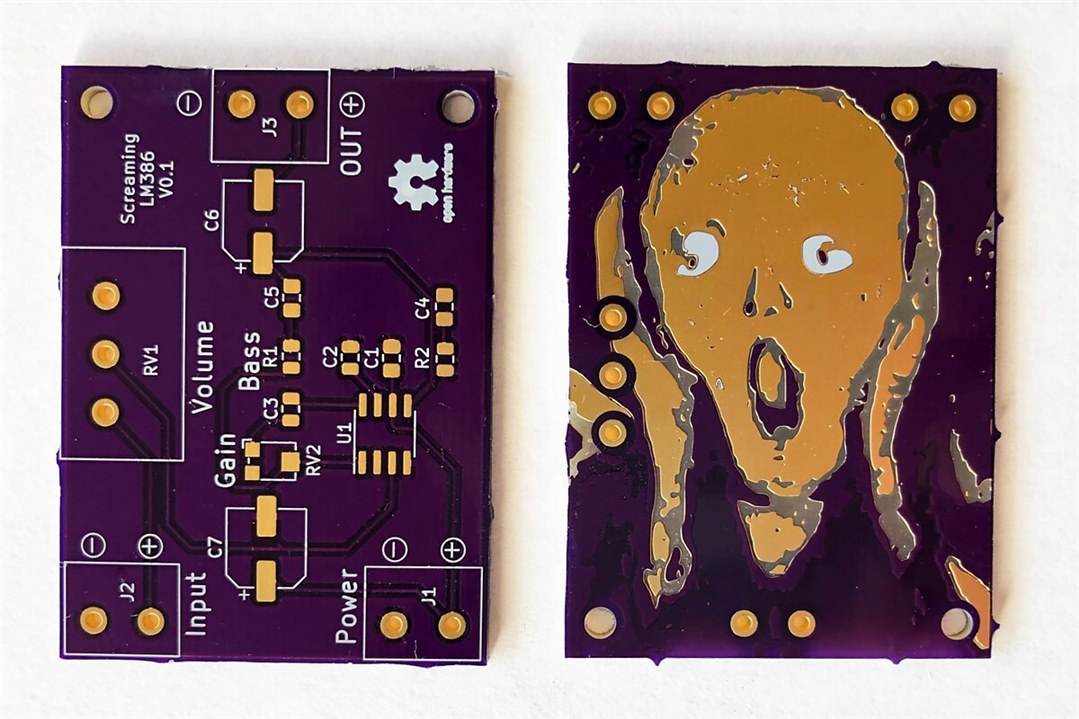The image depicts a purple circuit board with intricate designs and labels, presented on a white background. The board is adorned with golden contact pads labeled with functions such as input, output, power, volume, and "screaming" - indicating it could be an audio device, specifically the LM386V1 version. The left side of the image shows the front of the circuit board, featuring detailed trace lines and multiple contact points. The right side displays the back of the circuit board, where an artistic rendering of Edvard Munch's "The Scream" has been created by exposing the underlying copper surface. This depiction includes the iconic figure with white eyes and hands clutching its face, surrounded by dotted patterns. Both the front and back are meticulously crafted, showing a blend of electronic design and artistic expression.